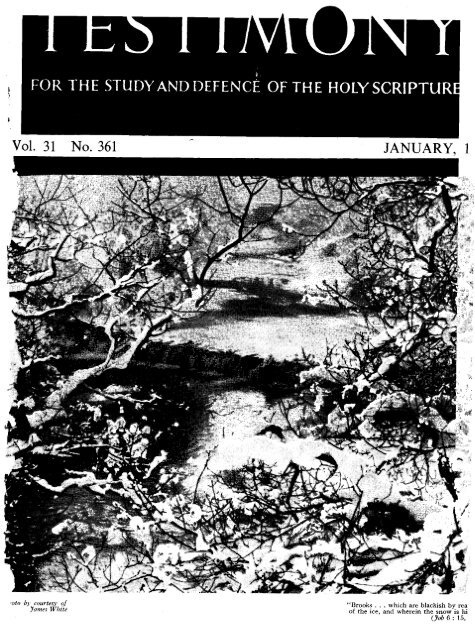The image appears to be the black and white, slightly damaged, photocopied cover of an old religious magazine. Across the top is a black banner with the white text, "Testimony for the Study and Defense of the Holy Scripture." Directly beneath is a thin white stripe with black text displaying, "Volume 31, No. 361," with the date, "January 1," visible on the right. The central part of the cover features a large black and white photograph covering over two-thirds of the page, depicting a barren desert-like setting with scrub brush and a stream or brook possibly covered in snow. There appears to be text at the bottom of the image that reads, "By Courtesy of Jonas White." A partially legible Bible verse is also present, likely referring to brooks and snow, though its exact phrasing is unclear due to the damage on the cover.